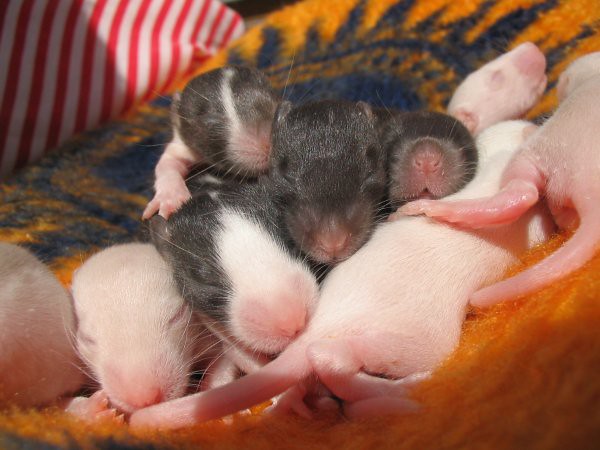The image captures a close-knit family of rats comfortably nestled together. At the center of the group is the sleeping mummy rat, characterized by her pure grey fur, with her head resting on the daddy rat, who is a dark grey and easily distinguishable by his large white nose. Surrounding the parents are at least eight to nine very small, baby rats. Most of the babies have pink, translucent skin at this stage, though one bears a resemblance to the parents with some grey coloring. They are all intertwined and snuggled up together in a tiny heap. The setting appears to be a small pet bed, which is primarily orange and black. In the background, you can also see a cushion adorned with red and white stripes. Overall, the baby rats' tiny pink paws, noses, and tails enhance the sense of their very young age. The cozy and warm ambiance of their nest is highlighted by the knitted blanket beneath them, colored in white with shades of deep yellow and navy blue trim.